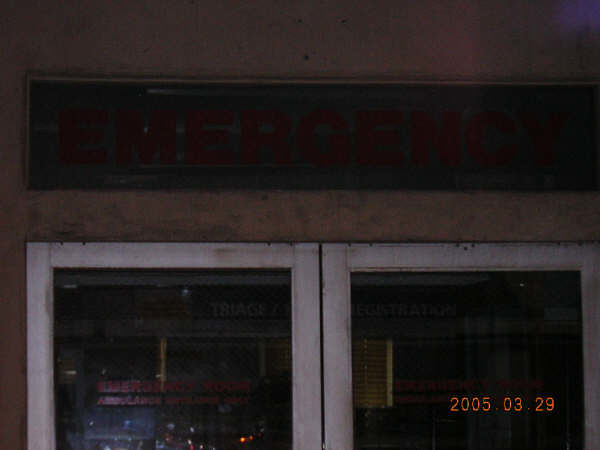This dark photograph captures the exterior of what appears to be an old, possibly abandoned hospital building, taken on a night in 2005 as indicated by the red digital date stamp in the lower right-hand corner, "2005-03-29." Above a set of white-framed, glass double doors is a sign that seems to read "EMERGENCY" or "EMERGENCIA," though the exact text is difficult to discern in the poor lighting. The building's facade features a mix of brown and black rectangles, adding to its dilapidated appearance. The doors, which show faint reflections of streetlights, suggest they might serve as an ambulance emergency entrance. The overall scene is shrouded in darkness, obscuring the fine details and making the image especially hard to analyze.